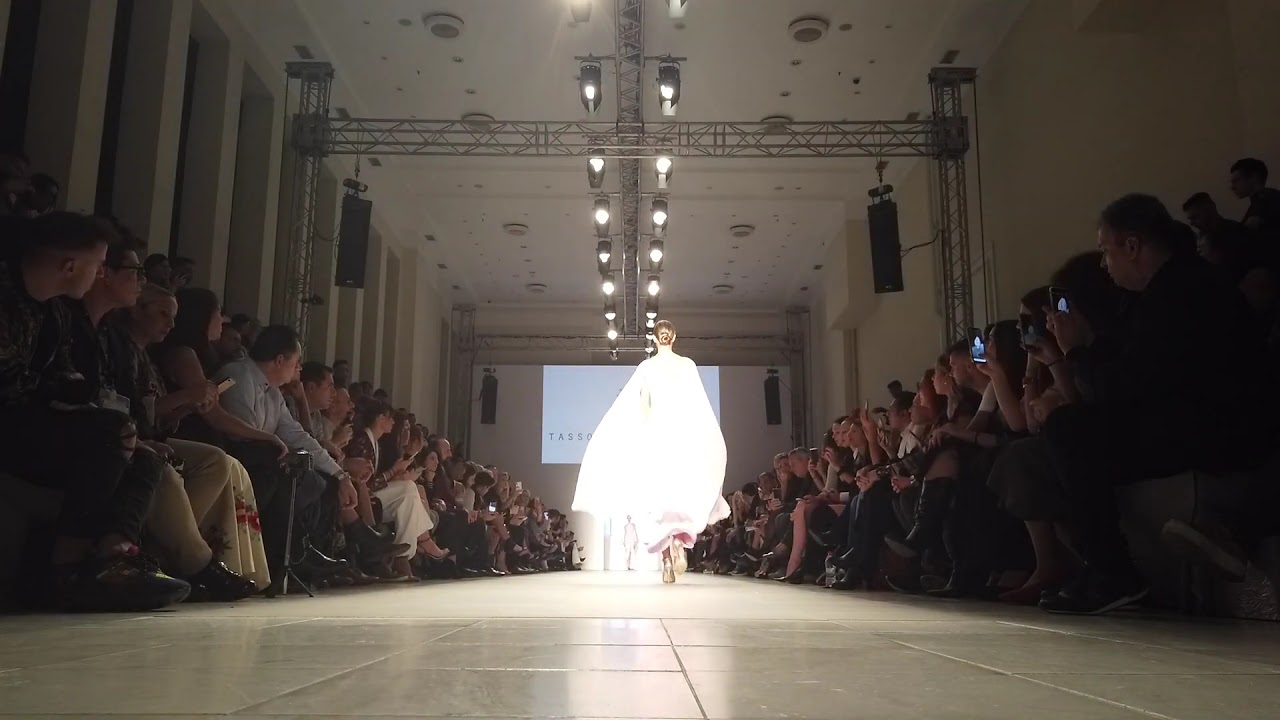In an indoor fashion show setting, a model elegantly walks down a long, narrow runway, adorned in a flowing, long white dress. The room, encased within white walls, is brightly lit by overhead lights, casting a radiant glow on both the model and her surroundings. The runway, a tan-colored tiled granite floor, guides the model towards a white screen at the far end of the room. Flanking the runway, three rows of spectators sit elbow to elbow on both sides, many capturing the moment with their cell phones and cameras. The scene is framed by black speakers hanging on the walls, adding an auditory backdrop to the visual spectacle. The intense focus of the onlookers, combined with the structured elegance of the setting, underscores the high fashion atmosphere of the event.